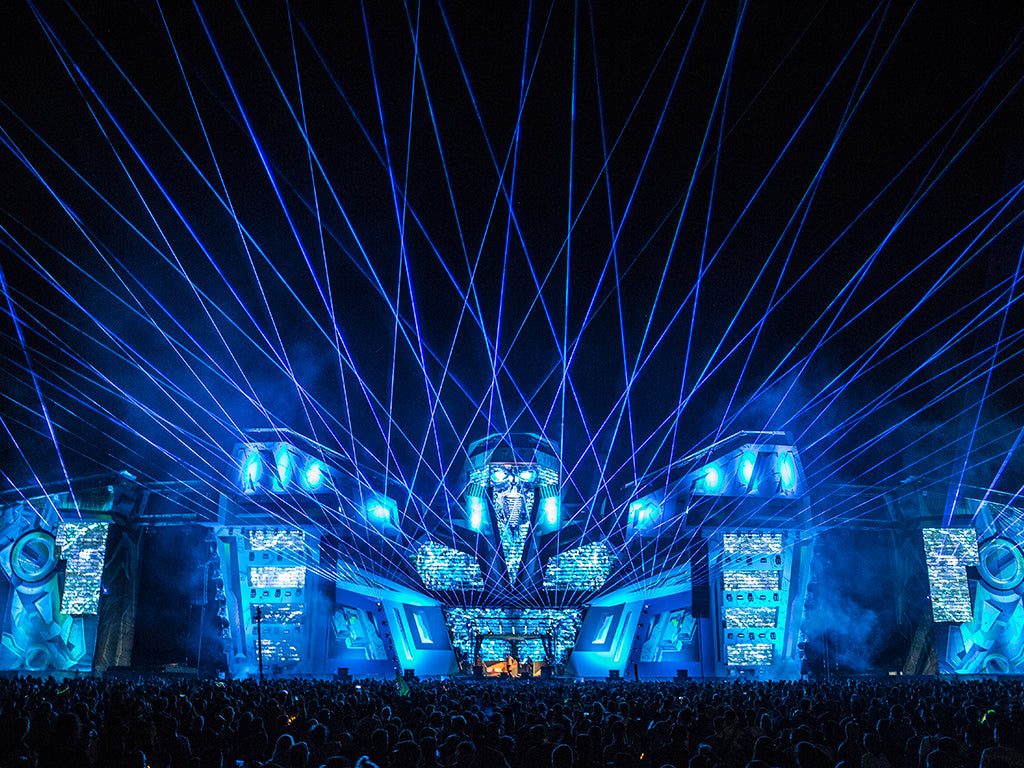In the image, a massive audience stands in front of an elaborate, expansive stage, bathed in hues of blue and dark blue. The stage features intricate constructions with metal inlets on either side and is adorned with light blue facades displaying some sort of imagery. Bright, purple lasers crisscross in all directions, with beams reaching far into the black night sky, forming an intricate grid of lines and shapes, including triangles, octagons, and circles. Spotlights from the grid illuminate the scene below, possibly highlighting a DJ on stage. The atmosphere is charged with energy as the crowd revels in the impressive laser show, creating a spectacular visual effect against the large structures and speakers, making it a night to remember.